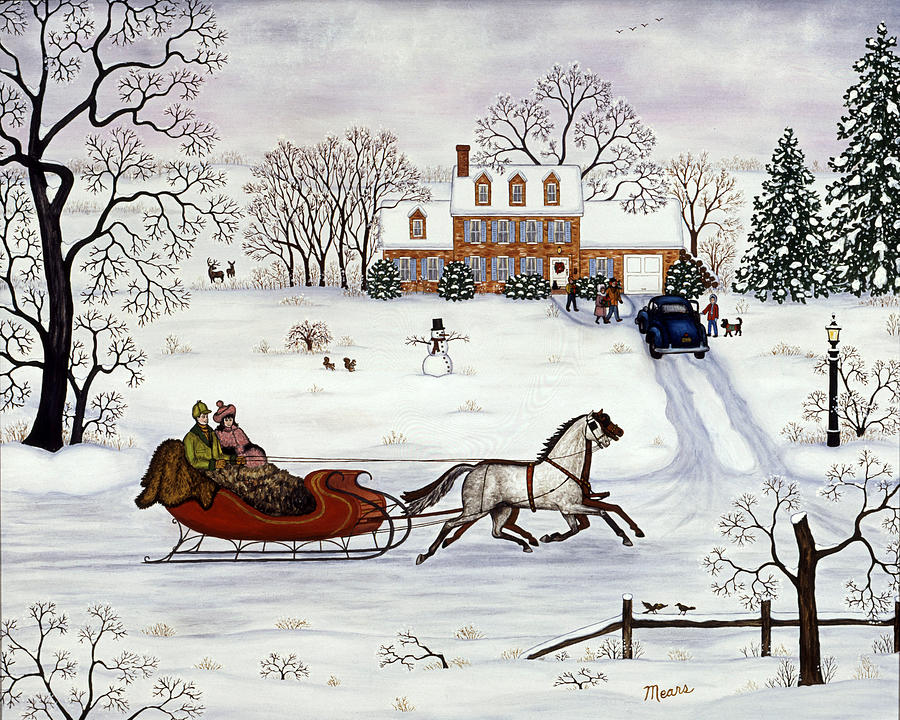This is a detailed painting or drawing depicting an idyllic winter scene, reminiscent of a traditional Christmas card. The scene is set against an overcast, white sky with snow blanketing the ground. Dominating the background is a large, orange brick, two-story house, complete with a driveway that cuts through the snow. The house features giant dormer windows on the top floor and multiple windows on the main part.

In the driveway, a vintage 1950s-style car is parked, suggesting the era of the scene. Nearby, family members, including a small dog, are either walking towards the car or waiting to greet arriving guests. A charming snowman stands proudly on the lawn.

In the foreground, a couple, warmly wrapped in blankets, enjoys a sleigh ride in an auburn-colored sleigh. The sleigh, pulled by a white and brown horse, moves from left to right down the snowy street. Additional details include a fence, a small tree in the immediate foreground, and two snow-covered pine trees to the far right. The serene, festive atmosphere captures the essence of a joyous holiday season.